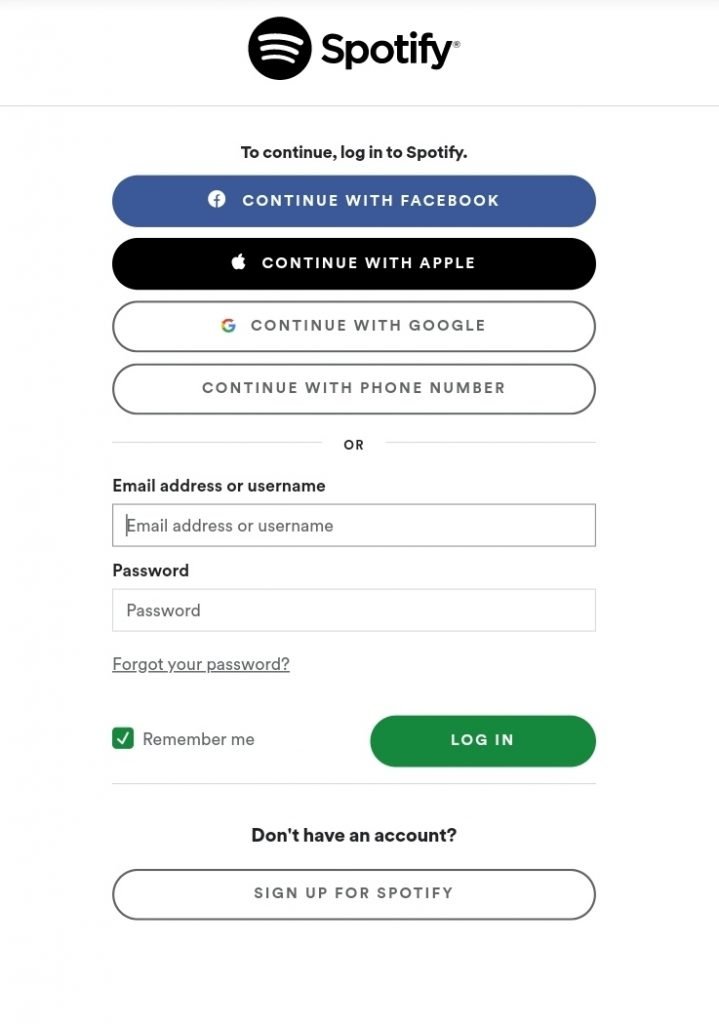The image depicts the login screen for Spotify. At the top, the Spotify logo is prominently displayed, followed by a prompt that reads "Continue to login to Spotify." Below this prompt, various login options are available:

1. A blue button labeled "Continue with Facebook."
2. A black button labeled "Continue with Apple."
3. A white button labeled "Continue with Google."

Following these options, there is an additional button labeled "Continue with phone number." Further down, there's a section to log in using an email address or username, accompanied by a text box for inputting the email or username, and another text box to enter a password. An "Forgot your password?" link, underlined for emphasis, is available beneath the password box.

Additionally, there is a checkbox labeled "Remember me" next to it, which is displayed with a green box and a checkmark. Below this, a green button prompts users to "Log In."

At the bottom of the screen, a message inquires, "Don't have an account?" followed by a white button that encourages new users to "Sign up for Spotify."